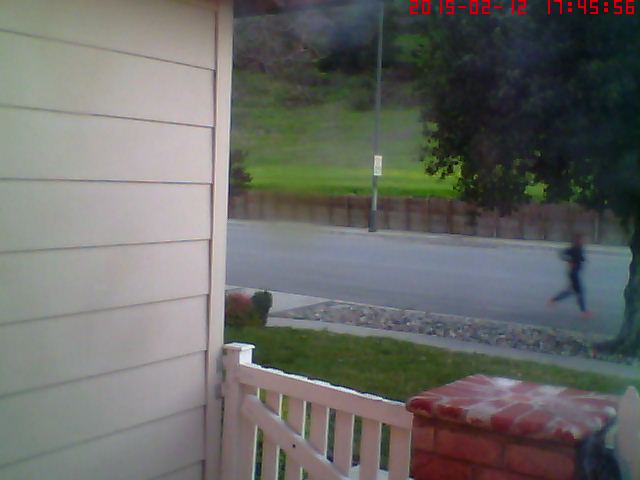The color photograph, likely taken from a front porch, captures a vibrant outdoor scene. To the left, the off-white, gray-shingled side of the house is visible, along with a white wooden gate at torso height, connected to a sturdy brick column. In front of the porch, a neatly maintained green lawn stretches outwards, punctuated by a single large tree near the sidewalk. The asphalt street beyond the lawn is dark gray, where a person, dressed in black attire and orange shoes, is caught in motion, appearing blurred due to their jogging. Further across the street, a concrete sidewalk lines up against a brown wooden fence, behind which lies an expansive green field dotted with wildflowers. A tall, gray cement post with a white sign stands prominently on the far side of the street, likely serving as a streetlight. The scene provides a detailed snapshot of a serene suburban neighborhood, blending natural elements with human activity.